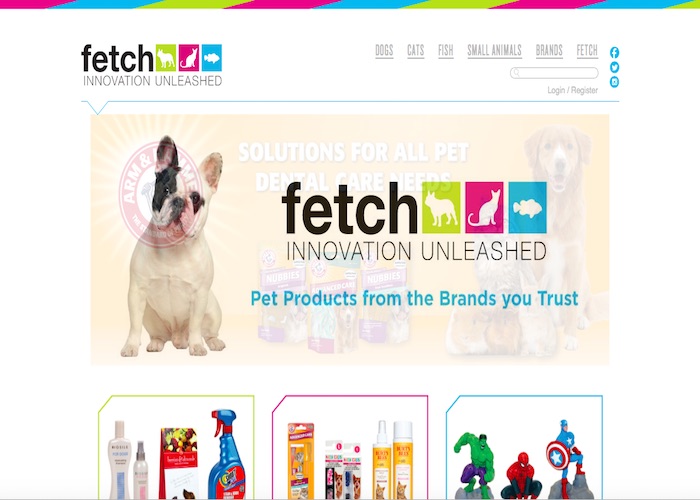### Screenshot of "Fetch Innovation Unleashed" - Online Pet Products Retailer

The screenshot showcases the website of an online company named "Fetch Innovation Unleashed," specializing in pet products. Central to the screen is the company's sizable logo, also replicated in the upper left corner. Adjacent to the primary logo are three distinct square icons: a green square featuring a white dog symbol, a magenta square with a white cat icon, and a blue square showing a small white fish symbol.

Beneath the logo, the tagline "Pet Products from the brands you trust" is prominently displayed. To the side, there's an image of a small bulldog-type dog, characterized by its white coat and black markings.

The upper menu bar offers several category options for navigation: Dogs, Cats, Fish, Small Animals, Brands, and Fetch. Further along the menu, three circular blue icons provide links to social media platforms, presumably Twitter, Facebook, and another social link. Adjacent to these icons is a search window, and below it, options for user login and registration, both shaded in gray.

A colored strip at the very top of the window features the company's three main colors: green, magenta, and blue, consistent with their branding.

At the bottom section of the screen, there are three clickable sections, each represented by a set of images. The first section with a green border highlights dog products, the second with a magenta border displays cat products, and the third with a blue border showcases fish products. Only parts of these sections are visible from the screenshot, indicating their focus based on the colored borders.

Overall, the website design is clean and user-friendly, allowing easy navigation across different pet product categories.